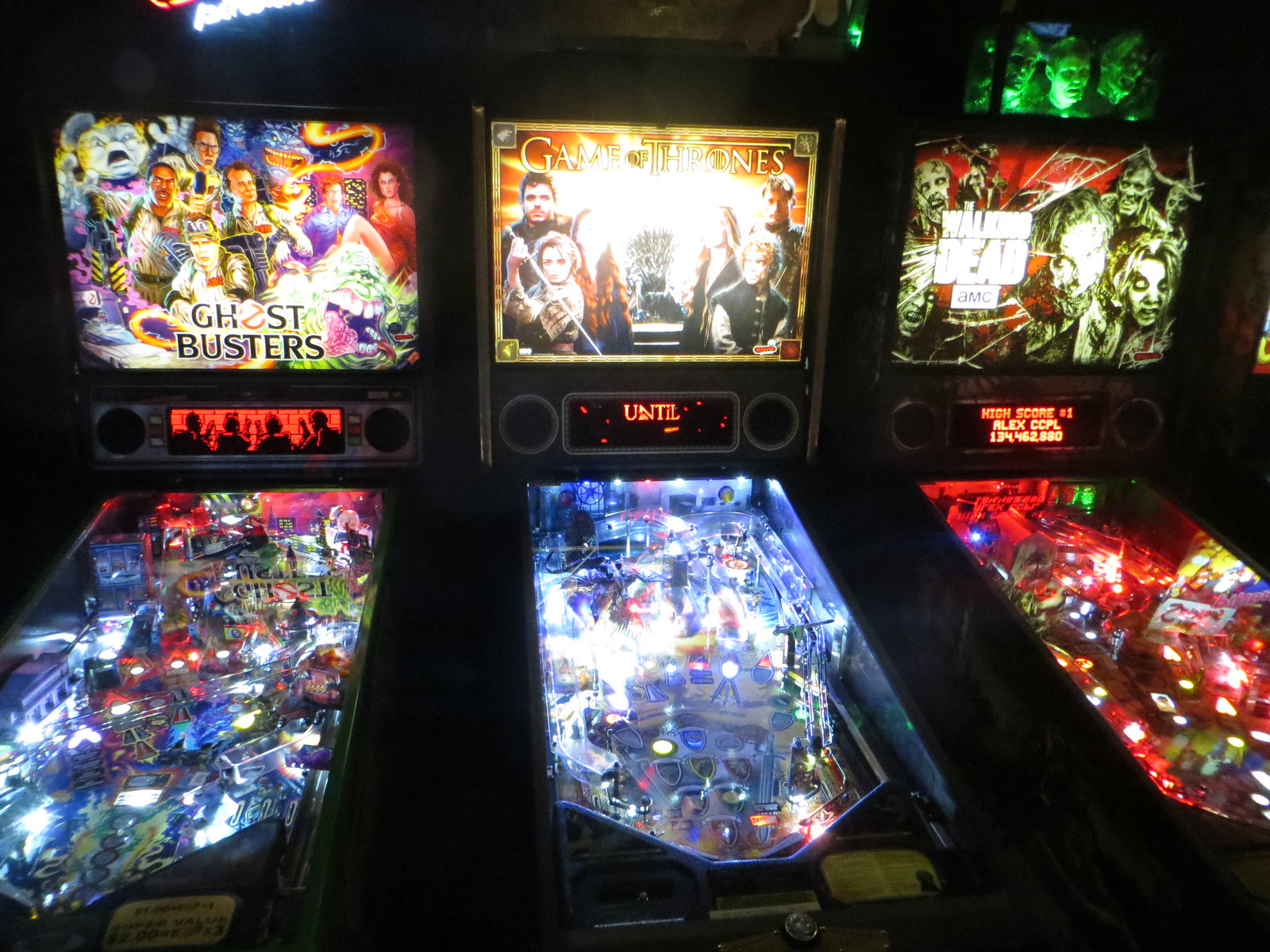This vibrant photograph captures the bustling atmosphere of a game arcade. Dominating the frame are three prominent game stations, each distinguished by its colorful and thematic graphics.

On the left, the iconic Ghostbusters game beckons players with its lively imagery, featuring the recognizable Ghostbusters logo and a montage of characters from the franchise. Bright hues of yellow, red, blue, and green make this station stand out vividly against the arcade's backdrop.

Centerstage is the Game of Thrones game, alluring fans with a detailed graphic that showcases prominent characters including Tyrion Lannister, Arya Stark, Jon Snow, and the formidable Iron Throne. The artwork is rich with the series’ signature elements, drawing players into the epic fantasy world.

To the right, The Walking Dead game station emanates an intense atmosphere with its theme of zombies. Dominating colors of red, black, and white create a haunting, post-apocalyptic scene, perfect for fans of the horror genre.

Beneath the visual feast, the display reads "High Score #1 Alex CCPL 1,134,462,880," commemorating an impressive achievement in one of these enticing games.